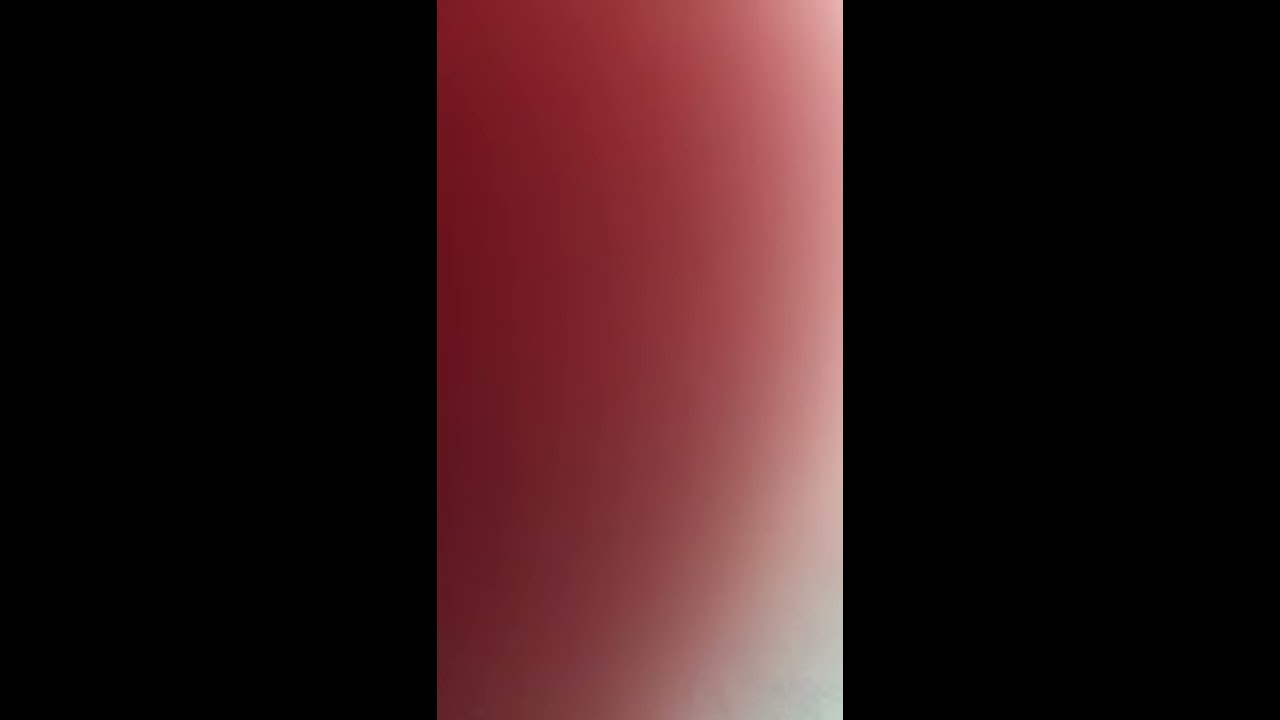This vertically-oriented image has black borders on the left and right sides, framing the scene. The core of the image is primarily a smooth, abstract composition dominated by a gradient transition from a flesh-tone pink or red on the left to a lighter, whitish area towards the right. The central part of the image features some distinct white vignetting, most prominently visible at the lower right and upper right corners. These lighter areas form irregular, almost triangular shapes. The image resembles an accidental close-up photograph where a finger is partially blocking the lens, resulting in a soft, blended color effect. The smooth transition and high-definition quality give the impression of a polished, minimalist aesthetic, evoking comparisons to content typically seen on social media platforms like Instagram or TikTok.